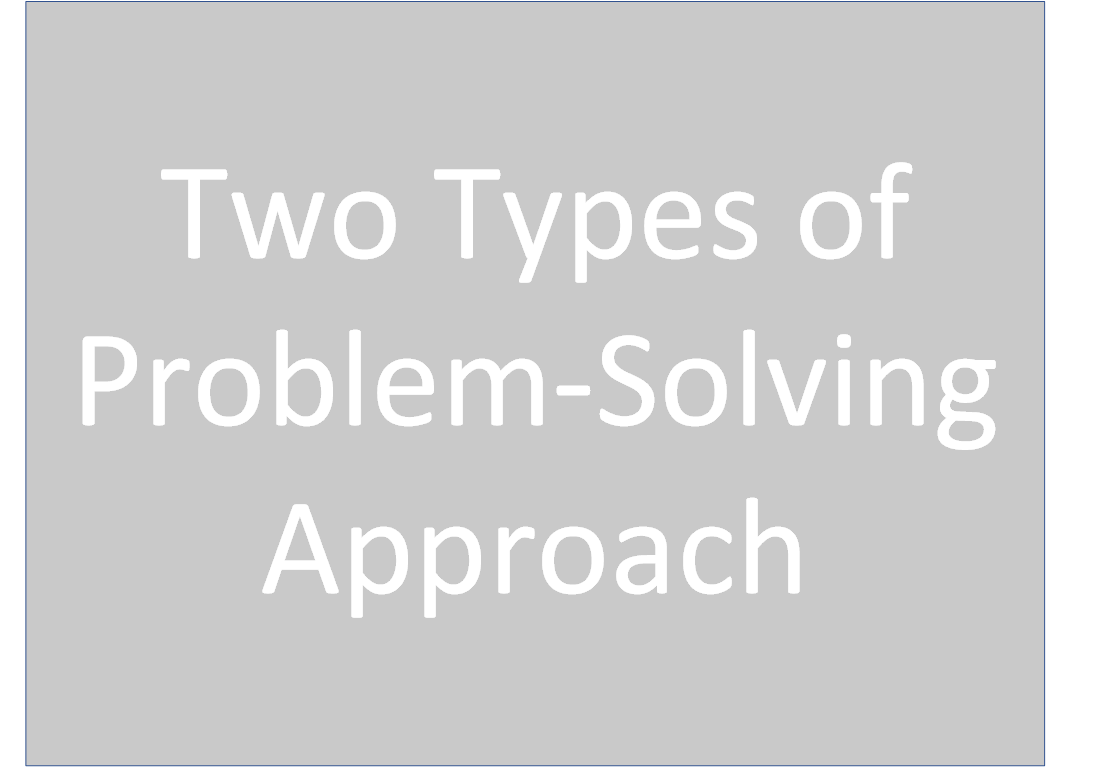The image features a plain grey background with a thin blue rectangular border. Centrally positioned on the grey background is a bold, white text spread across three lines, reading: "Two types of problem-solving approach." The text is large and prominently displayed, emphasizing that there are two methodologies for tackling problems. The phrase "problem-solving" includes a hyphen. The image is minimalist, containing no other elements or punctuation beyond the described text.